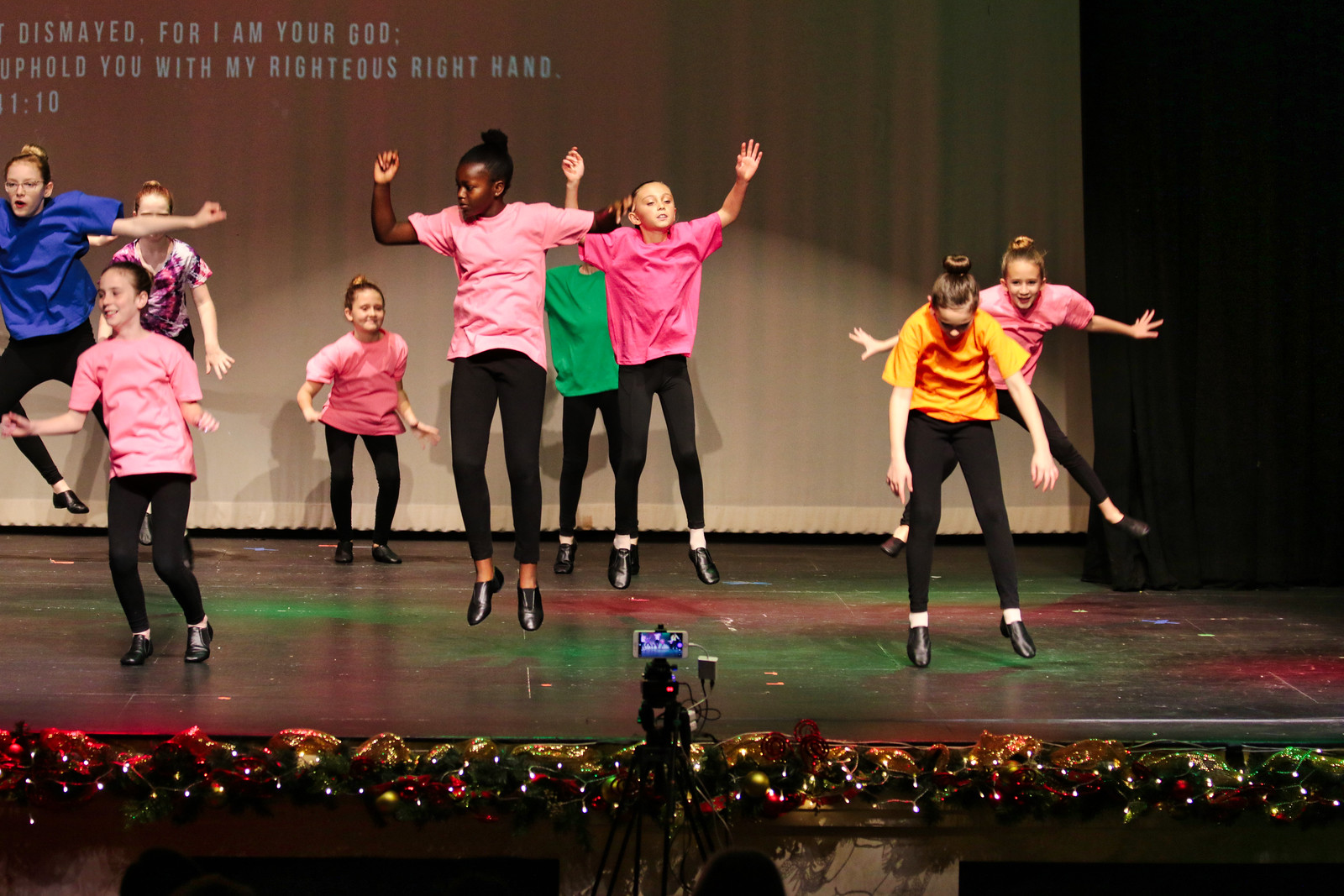In this image, several young girls, all between the ages of approximately 7 to 12, can be seen on a stage in an auditorium, evidently performing a dance or participating in a play. They are all wearing black shoes and black tights, paired with brightly colored shirts in shades of blue, green, white, pink, dark pink, and yellow. The diverse group primarily consists of Caucasian girls, but there are one or two African American girls among them. Centered on the stage, they appear to be the focal point of the performance.

The stage is adorned with festive Christmas decorations, indicating a holiday-themed event. At the bottom of the image, a camera is visibly set up, capturing the performance, and in front of it, the back of someone's head is also noticeable. On the top left against the back wall, a partially visible Bible verse reads, "Dismayed, for I am your God, uphold you with my righteous right hand," though the rest of the text is cut off. The indoor setting of the image and the nature of the event suggest it takes place during some type of school or community performance.